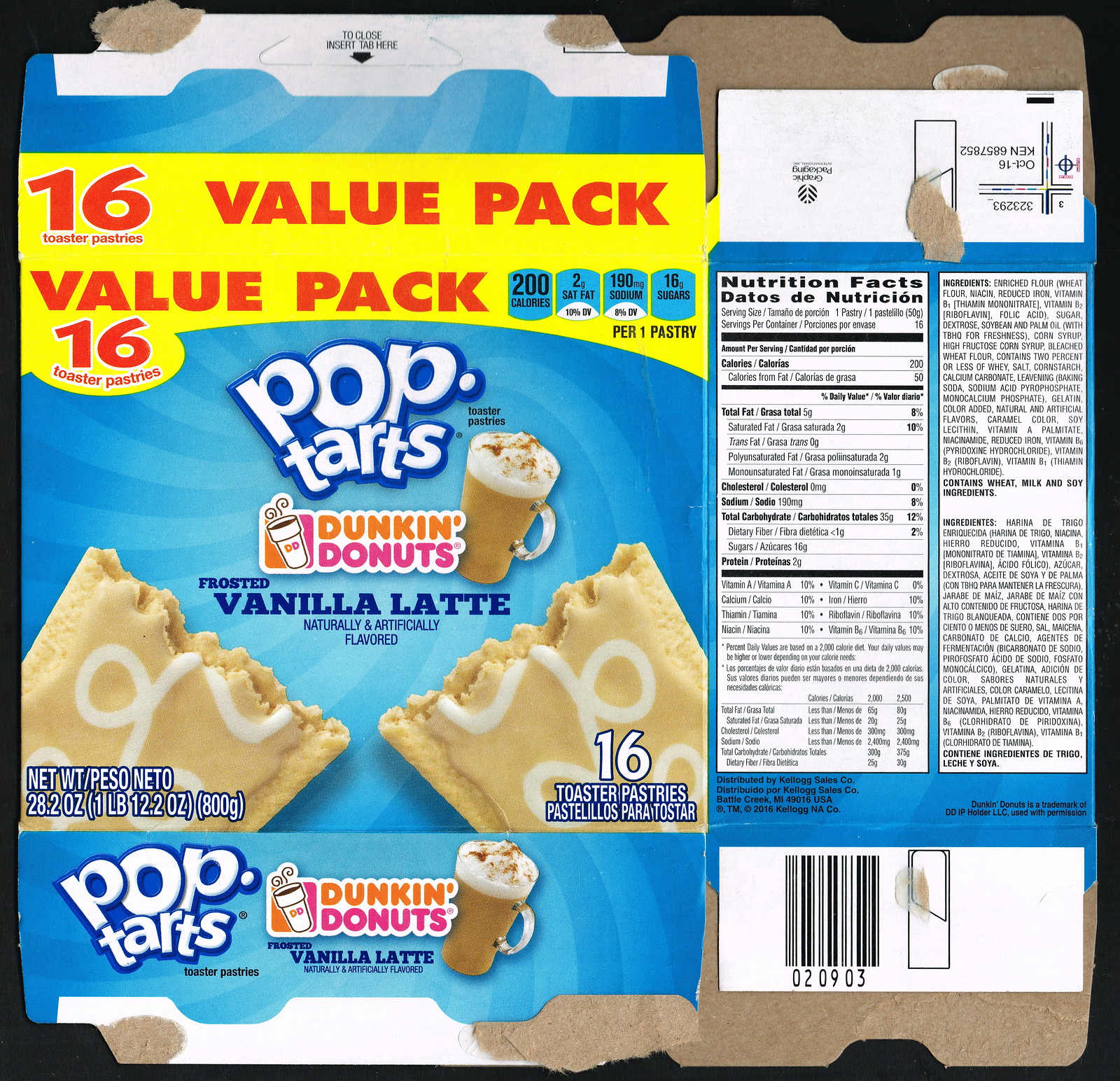This detailed photograph features a fully flattened box of Pop-Tarts. Predominantly blue, the box prominently displays a yellow band near the top, emblazoned with the text "16 Value Pack, Value Pack 16." Directly below this band, the iconic Pop-Tarts logo is visible, followed by the Dunkin' Donuts branding, complete with the distinctive orange and pink Dunkin' Donuts logo that includes a coffee cup illustration.

The flavor, "Frosted Vanilla Latte," is prominently showcased, along with an image of two tan-colored Pop-Tarts adorned with swirly white frosting. Near the bottom of the box, the Pop-Tarts and Dunkin' Donuts branding is reiterated, along with the specific flavor name, "Vanilla Latte." On the right side of the box, various product details are displayed, including the Nutrition Facts and the Ingredients List. A barcode is situated at the bottom right corner of the flattened box.

The entire box is set against a black background, which effectively frames and highlights it, creating a stark contrast that draws attention to the vibrant packaging details.